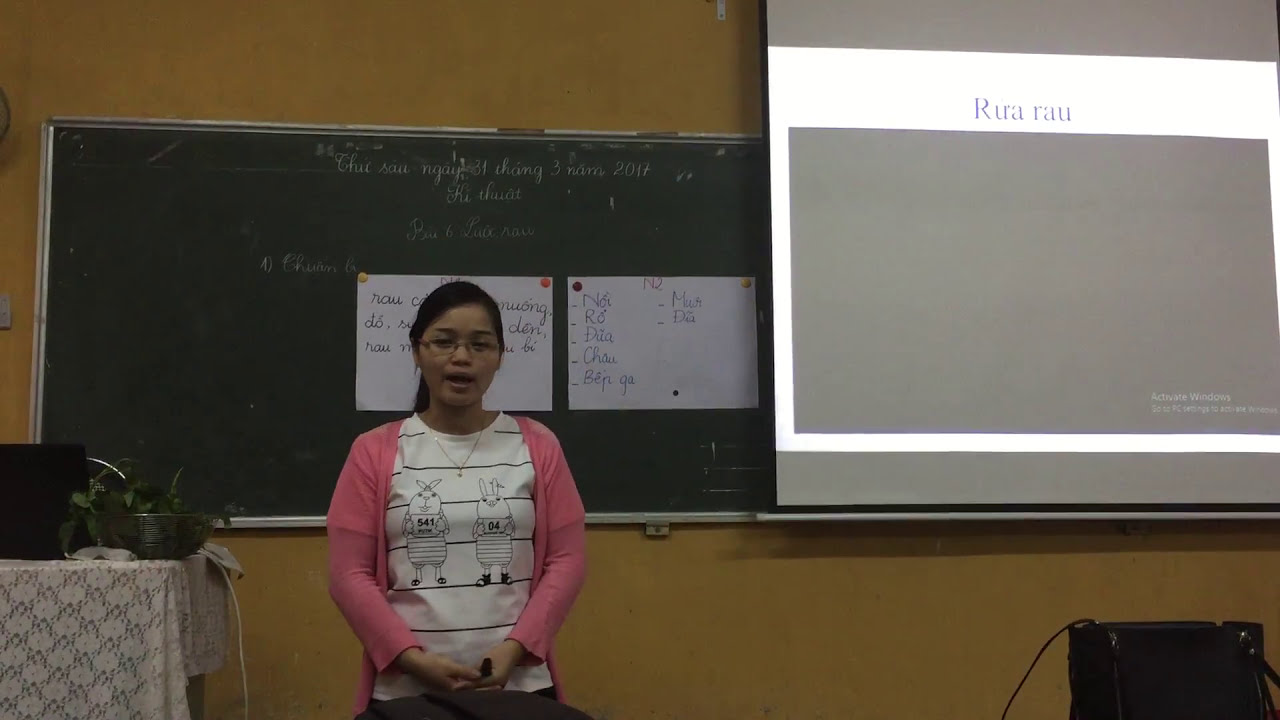This photograph captures a detailed scene of a classroom setting. The focal point is a young Asian woman standing at the front of the room, directly facing the viewers. She has black hair tied in a ponytail, wears glasses, and her mouth is open as she appears to be teaching. The woman is dressed in a white shirt adorned with illustrations of cartoon animals, a pink cardigan, and blue jeans; her hands are clasped in front of her.

The classroom has a yellow wall that features a green chalkboard and a display screen. On the chalkboard, written in Vietnamese, is some text, along with two white pieces of paper that are either magnetized or clipped to it. The display screen next to the chalkboard shows a slide with additional Vietnamese text and a large, rectangular black box. 

To the left of the woman, there is a table covered with a lace tablecloth. On the table, a potted plant and various other items, including a black box, are neatly arranged. A black purse rests at the bottom right corner of the picture, completing the scene.